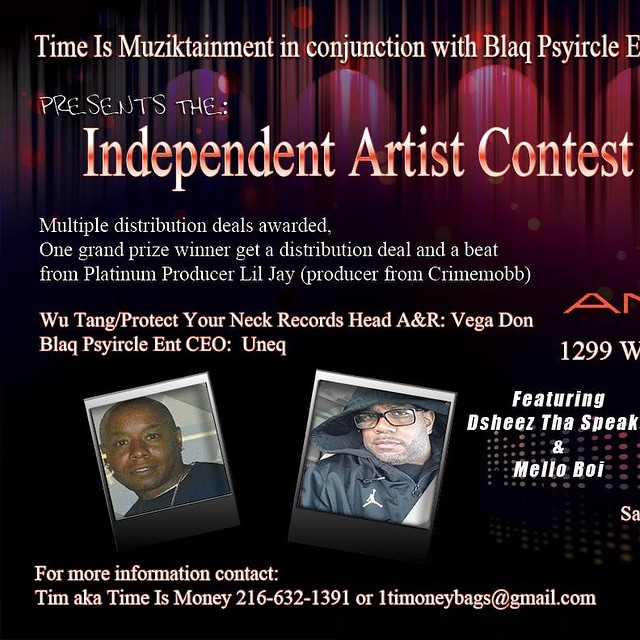This image is a party flyer featuring a dark stage background. At the top, it reads "Time is Musictainment" in conjunction with "BLAQPSYIRCLE." The flyer announces "The Independent Artist Contest," highlighting that multiple distribution deals will be awarded. Additionally, one grand prize winner will receive a distribution deal and a beat from Platinum producer Lil Jay, a producer from Crime Mob. The flyer also mentions "Wu-Tang/Protect Ya Neck Records" with Head A&R Vega Dawn and "Black Cyrcle Entertainment" CEO Unique. Two black men are pictured at the center of the flyer. To the right of their photos, it features artists "D-Sheez Tha Speak" and "Mellow Boy." For more information, the flyer provides contact details: Tim, aka Time is Money, at 216-632-1391 or via email at 1timoneybags@gmail.com.